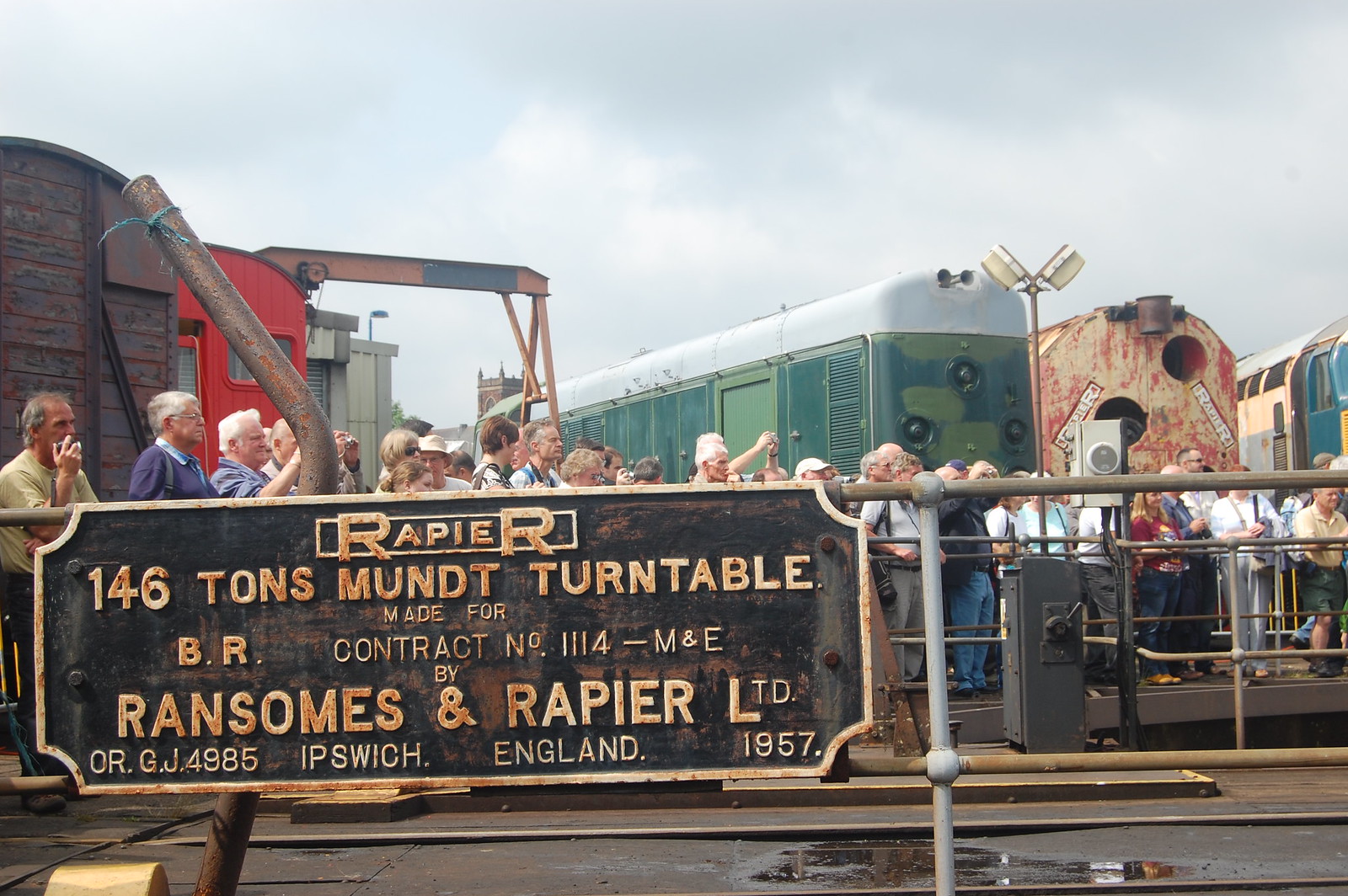In the foreground of a weathered train yard, a rusted metal barrier fashioned from what were once silver pipes stands prominently. The barrier, consisting of a top pipe and another midway down, is anchored into the ground. Attached to the left end of this barrier is a severely rusted sign with a black background and faded yellow and orange text. The sign reads: "Rapier, 146 ton mundant turntable, made for BR contract number 1114-M&E, Ransoms and Rapier Ltd, ORJJ 4985, Ipswich, England, 1957."

Behind this barrier stands a large group of 30 to 50 mostly elderly, Caucasian people, their faces turned to the right as if observing something out of shot. Scattered within the group are individuals holding up cameras. The sky above is filled with gray and white clouds, hinting at recent rain, evidenced by a small puddle in the foreground.

Through the barrier and past the crowd, several old train cars are visible, each bearing the wear of decades. The central car is distinctly colored with a green base, blue bottom, and white top. To its front, a utility pole with white lights extends, with one light pointing down to the left and another to the right. Other train cars in the background display a palette of colors including brown, red, pale green, bright green, yellow, and blue, all showing signs of age and rust.